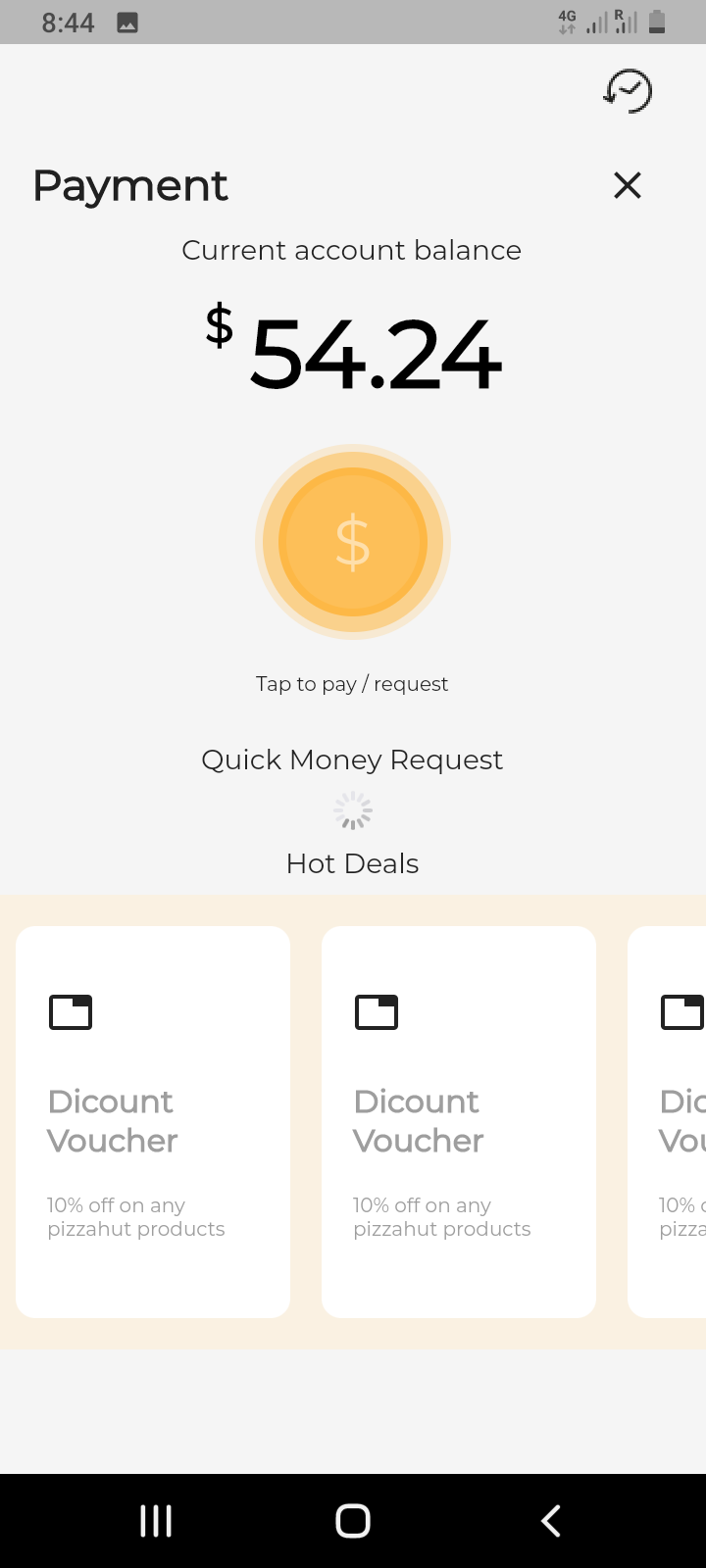Screenshot of a Mobile Payment Interface

At the top of the screenshot, several status icons are visible, indicating time, network connection, Wi-Fi connection, and battery life. Along the bottom of the screen, three icons on a black background are displayed: three vertical lines (menu), a square (home), and a backwards arrow (back).

The main content of the screenshot features a light grey background. At the top, in bold black text, the word "Payment" is prominently displayed. Below this heading, the current account balance is shown as $54.24. An orange-yellow circle containing a white dollar sign is positioned beneath the balance, accompanied by an instruction to "tap to pay/request."

Further down, a scrolling carousel-style menu showcases discount vouchers. Notably, the word "discount" is misspelled as "D-I-C-O-U-N-T." The vouchers offer a 10% discount on any Pizza Hut products.